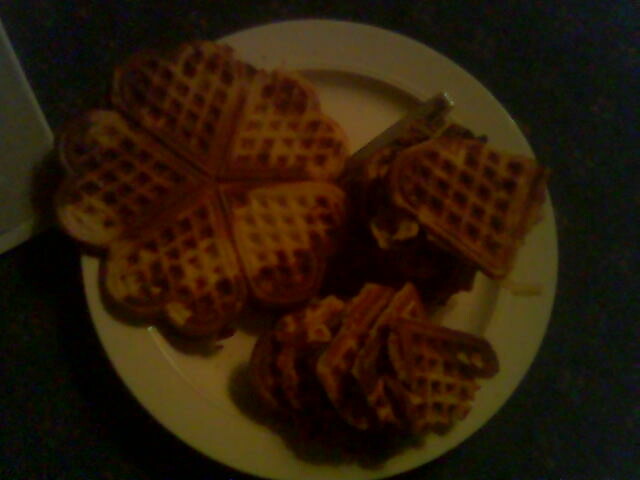In this dimly lit photograph, a white, circular plate sits on a black granite countertop, displaying what appear to be cooked, frozen waffles. The focal point of the image is a unique waffle design, where five heart-shaped sections are connected to form a circular, clover-like pattern. Among the waffles, some are whole, while others are broken or half-eaten, with one complete clover-shaped waffle prominently positioned on the left side. The waffles are drizzled with syrup, which pools in certain areas, giving a dark, glossy appearance. A metallic object, possibly a fork, is faintly visible on the right side of the plate, adding a subtle detail to this otherwise shadowy scene.